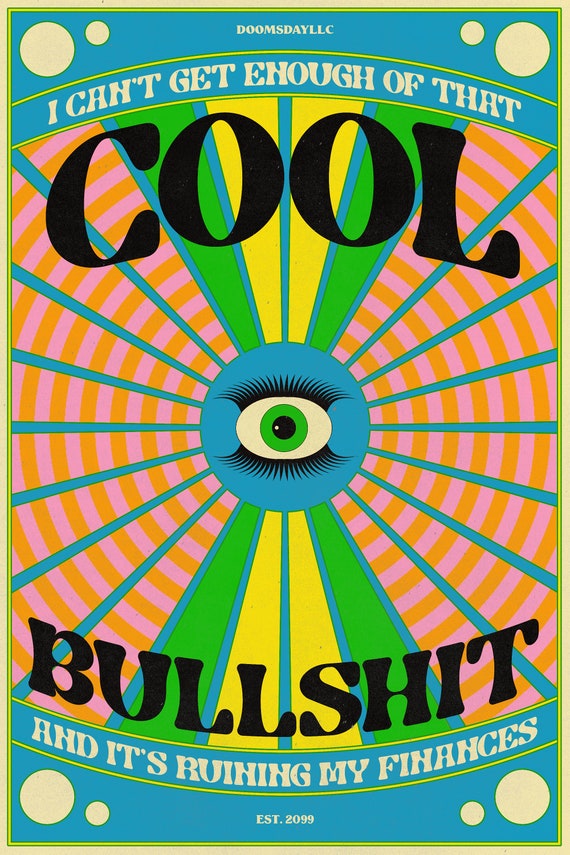This is a highly detailed and psychedelic poster with a retro 1970s style, reminiscent of old-school Grateful Dead concert art. At the top of the poster, bold text reads "Doomsday LLC" and "I can't get enough of that cool bullshit," while the bottom has "and it's running through my finances" and "Established 2099". The central focal point is a large, peculiar eye with exaggerated, almost alien-like eyelashes both above and below the eye. Surrounding the eye is a psychedelic sunburst design, with blue rays emanating from the center, interspersed with hypnotic rings of pink, light red, and orange. These rays are detailed with segments in vibrant yellow and green, creating an intricate and colorful pattern. The text is primarily blue, complemented by small white circles in the corners, adding to the poster's overall trippy and abstract aesthetic.